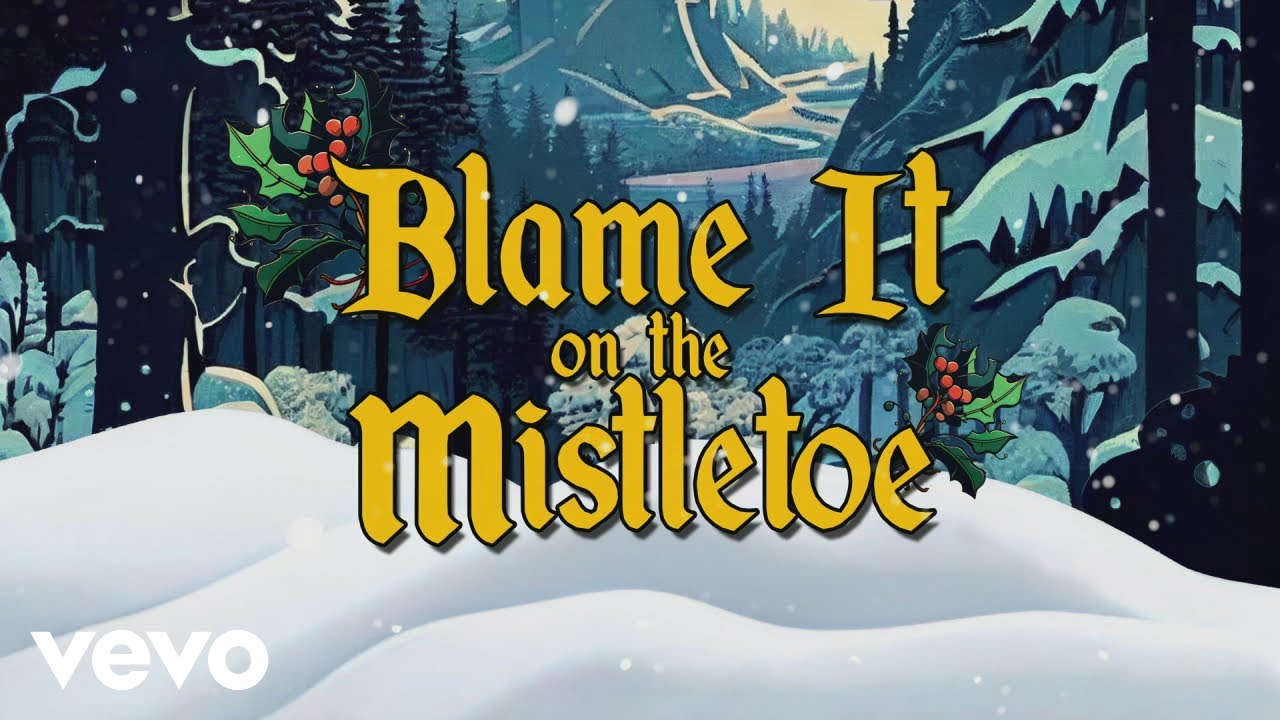The image is a screenshot from a TV episode, cartoon, or movie that features a winter scene. Dominating the center of the image is large, stylized yellow text that reads, "Blame it on the Mistletoe," with sprigs of mistletoe cleverly placed on the letters 'B' and the last 'E'. The bottom left corner displays the logo "VEVO," a video-sharing company. The background showcases a picturesque landscape with snow-covered conifer trees, a snowbank stretching across the image, a serene river, and a majestic snow-capped mountain. Snow is softly falling, adding to the tranquil and festive atmosphere. No characters are visible in this serene and snowy scene.